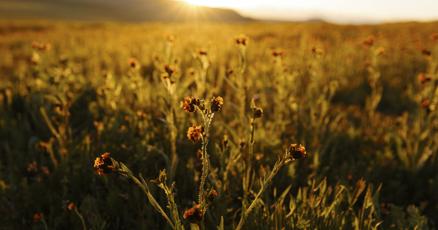In this captivating nature photograph taken during either sunrise or sunset, a vast field extends towards the horizon and is densely populated with green plants that appear to be adorned with thorns and capped by pink flowers. The sun sits low on the horizon, casting a warm, glowing light across the landscape, with the underexposed lower areas of the field creating a vivid contrast. The sunlight bathes the plants in vibrant hues, illuminating them like a fiery tapestry. Despite some ambiguity about the exact type of vegetation, it closely resembles the weed known as Stinging Meadow, common in regions like Kansas and the Midwest. In the distance, a dark hill or mountain looms against the sky, adding depth to the scene and enhancing the natural beauty captured in this moment.